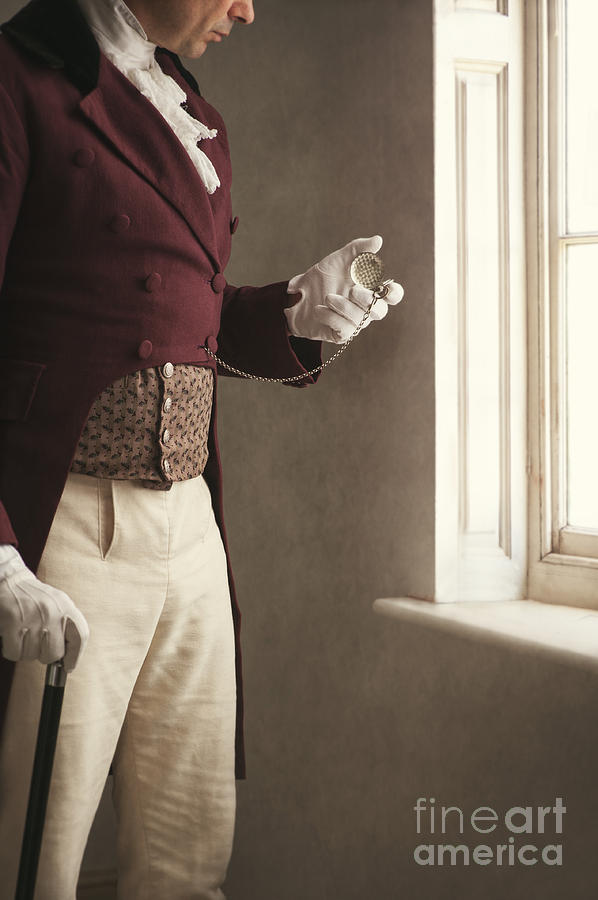In this evocative photograph labeled "Fine Art America" in the bottom right corner, a white gentleman is depicted in an old-timey, perhaps colonial, attire. He stands in profile within a white room, near the frame of a window that allows sunlight to filter in. Only his face from his nose down is visible. He is adorned in a frilly white shirt underneath a burgundy red, buttoned jacket that opens slightly at the midsection, revealing a beige cummerbund with four buttons. Complementing his ensemble, he wears khaki pants and white gloves. In his right hand, he clutches a black cane, while his left hand is elevated, carefully examining a pocket watch attached by a chain to his blazer. The intricate details of his attire and the serene ambiance of the white room combine to create a finely detailed and period-specific portrait.